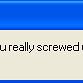The image depicts a very small, close-up snippet of what appears to be a message on an older computer interface. The top of the screen is colored dark blue, and the message text beneath it is rendered in a black font against a beige background. Only a fragment of the message is visible, showing the words "You Really Screwed?" with text potentially being cut off from a longer phrase such as "You Really Screwed Up?" The entire image is surrounded by an empty, white background, giving the impression of isolation and starkness. The scene is reminiscent of an old Instant Messenger or program notification, though the specific details about the program or sender are absent due to the cut-off nature of the image.